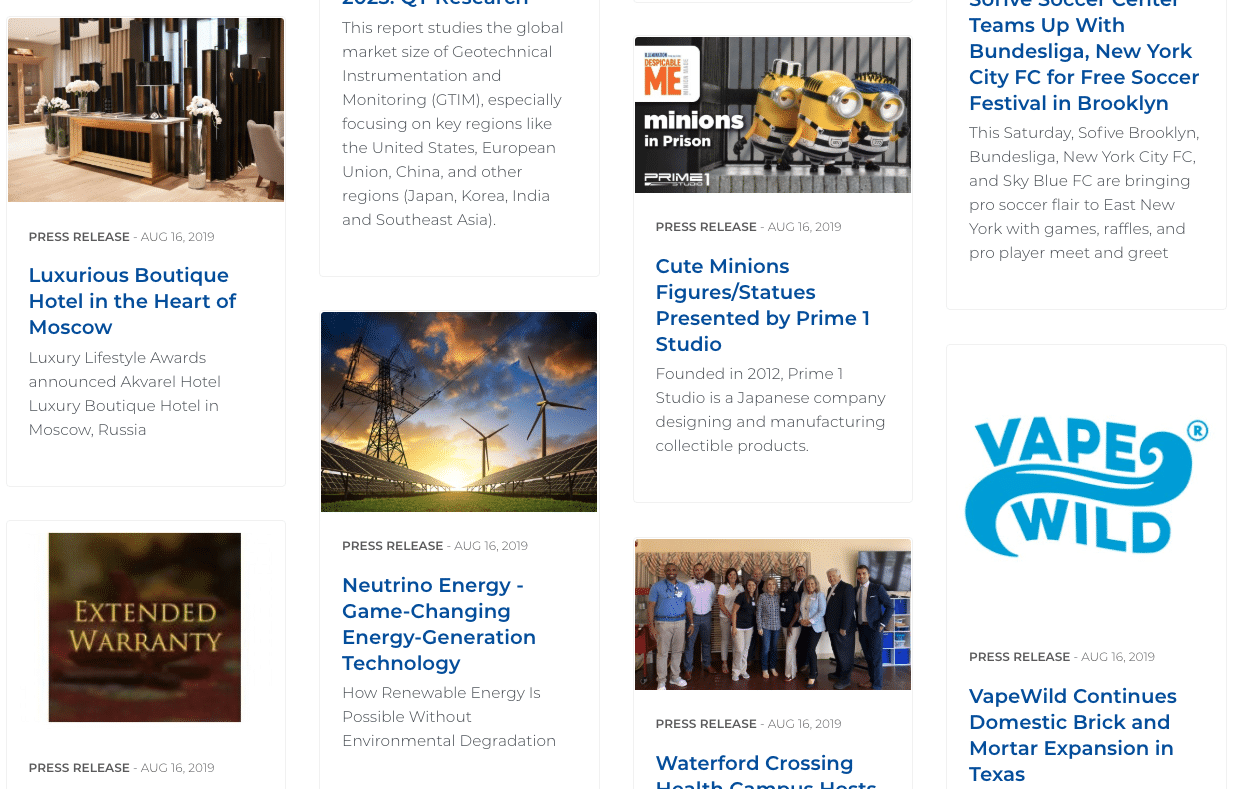This image displays a collection of clickable articles, each labeled with a "Press Release" tag followed by a date and an introductory paragraph summarizing the content. At the top of the image, a press release from August 16th, 2019, announces the opening of a luxurious boutique hotel in the heart of Moscow. Below, a cropped article titled "Extended Warranty" is visible.

Positioned above is another article that examines the global market size of geotechnical instrumentation and monitoring, with a particular focus on key regions such as the United States and the European Union. Adjacent is a press release dated August 16th, 2019, featuring an image of windmills alongside a text detailing Nutrimo Energy's groundbreaking energy generation technology.

The image also includes an article showcasing cute Minions figures and statues presented by Prime 1 Studio. Further down, a partially visible press release discusses Waterford Crossing, while another snippet mentions Vape Wild. Lastly, there is a reference to a free soccer festival taking place in Brooklyn.